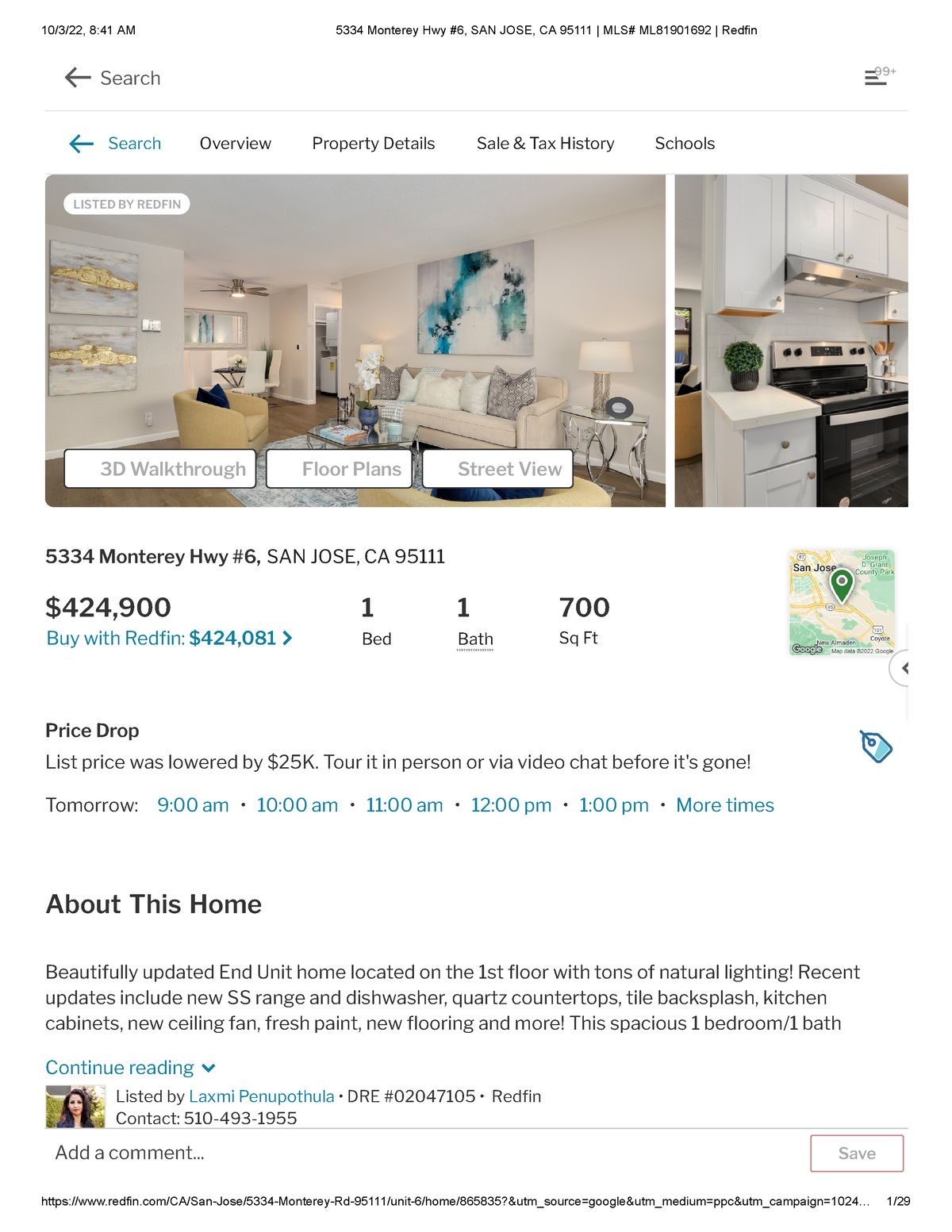This image captures a screenshot of a real estate listing on a website. At the top, there's a date in small font, reading "10.3.10.3.22, derived at 8:41 AM," followed by an address: "5334 Monterey, #6, San Jose, CA 9511." Below, the listing number is displayed as "MLS# ML81901692," accompanied by the Redfin logo.

Underneath these details, there's a search bar with an arrow pointing to the left. The navigation menu includes "Overview," "Property Details," "Sale & Tax History," and "Schools."

The central part of the screenshot features two images: one of an indoor living room with wooden floors, white walls adorned with abstract art, white couches, and a sliver of an adjoining kitchen on the right. The kitchen is partially visible.

Below the photos, the address "5334 Monterey, #6, San Jose, CA 9511" is repeated, followed by the listing price of "$424,900." The phrase "Buy with Redfin: $424,081" appears underneath.

Further details provide the property specs: one bedroom, one bathroom, and 700 square feet. A small map to the right shows the property's location. Additionally, there's a note about a recent price drop of $25K, with a prompt to "Tour in person or via video chat before it's gone!" with available times listed as clickable links (9:00 AM, 10:00 AM, 11:00 AM, 12:00 PM, 1:00 PM, and more).

The "About This Home" section, highlighted in bold, describes the property as "Beautifully updated in-unit home located on the first floor with tons of natural lighting!" Recent upgrades include a new stainless steel range and dishwasher, quartz countertops, tile backsplash, kitchen cabinets, new ceiling fan, fresh paint, new flooring, and more. Below this description, there's a "Continue Reading" option.

An image of a woman with light skin and brown hair is shown with the caption "Listed by," followed by a contact number: 510-493-1955. Finally, to the right, there's a comment section and a "Save" button.